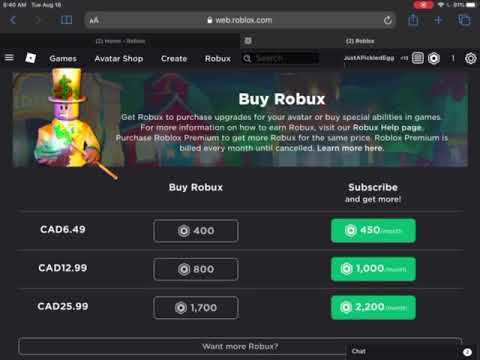This image is a detailed screenshot from the Roblox website, specifically the web.roblox.com interface. At the top of the screen, the navigation options include "Games," "Avatar Shop," "Create," and "Robux." The username displayed is "Just a Pickled Egg."

The focal point of the cartoon illustration features a character drawn in a simplistic, yet eye-catching style. The character is donned in a luxurious gold top hat adorned with green dollar signs and a matching gold-colored tuxedo, exuding an aura of wealth. He holds a sizable stack of money in his right hand while his left hand wields a wand topped with a glowing green money sign, seemingly enchanting or interacting with the money.

To the right of the cartoon, there is a prominently highlighted section for purchasing Robux, the virtual currency used for various upgrades and special abilities in the game. Detailed descriptions inform users about the benefits of buying Robux or subscribing to Roblox Premium for more value. The pricing is listed as follows:

- CAD $6.49 for 400 Robux (450 on subscription)
- CAD $12.99 for 800 Robux (1000 on subscription)
- CAD $25.99 for 1700 Robux (2200 on subscription)

Additionally, the screen advises users to visit the Robux Help page for more information on earning Robux and highlights that Roblox Premium is billed monthly until canceled.

At the bottom of the screenshot, there is a chat window option, indicating a space for user interactions and support.